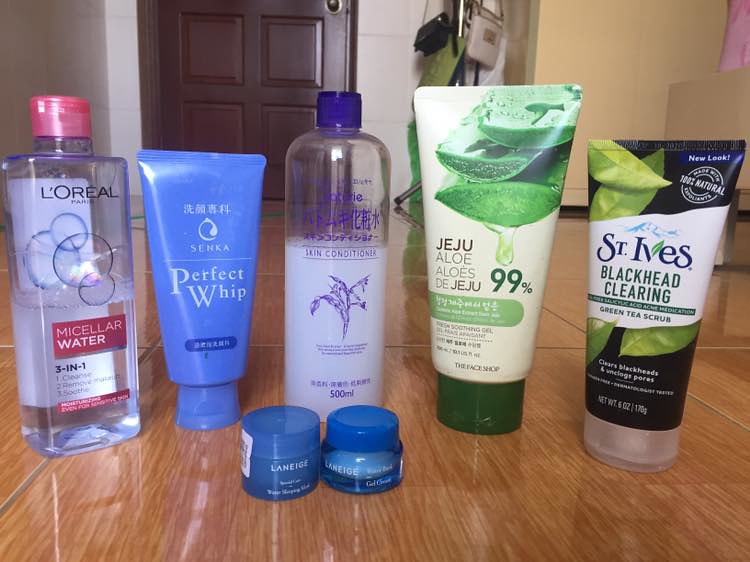This image captures an array of skincare products neatly arranged on a highly polished wooden tile floor, which reflects the items due to its shiny surface. In the background, a dark brown paneled wooden door stands prominently. To the right of the door, there's a coat rack adorned with several purses, hinting at a functional and stylish organizational setup. Further to the right of the coat rack, part of a white bathtub is visible, indicating that the photograph was taken in a bathroom setting.

From left to right, the skincare collection includes:

1. **L'Oreal Paris Micellar Water 3-in-1**: A translucent bottle with a pink lid, marked with the functions of cleansing, makeup removal, and soothing. The label's text is partially readable, but the volume is not specified.
   
2. **Senka Perfect Whip**: A smaller, upside-down lotion bottle in periwinkle blue, featuring Japanese text and the brand's name in English.

3. **Saptoree Skin Conditioner**: A larger, shampoo-sized, translucent bottle with a purple lid. It bears the brand name in purple text, alongside Korean characters. The bottle's content is 500 milliliters and includes an image of a plant.

4. **Two Small Blue Bottles**: Positioned in front of the larger bottles, these medium blue containers with matching blue lids resemble slightly oversized contact lens cases.

5. **Jeju Aloe Lotion**: A notable white bottle representing a larger size within the collection, featuring aloe imagery and partially readable French text "Jeju aloe, aloes de Jeju, 99%". The rest of the details are obscured.

6. **St. Ives Blackhead Clearing Green Tea Scrub**: A distinct black bottle adorned with green leaves. The label highlights it as a "New look" product, emphasizing its natural quality. The scrub claims to clear blackheads and unclog pores, with a net weight of 6 ounces or 170 grams.

Overall, the arrangement of skincare products on the bathroom floor offers a glimpse into a curated beauty routine, showcasing a range of international brands and product types used by the individual.